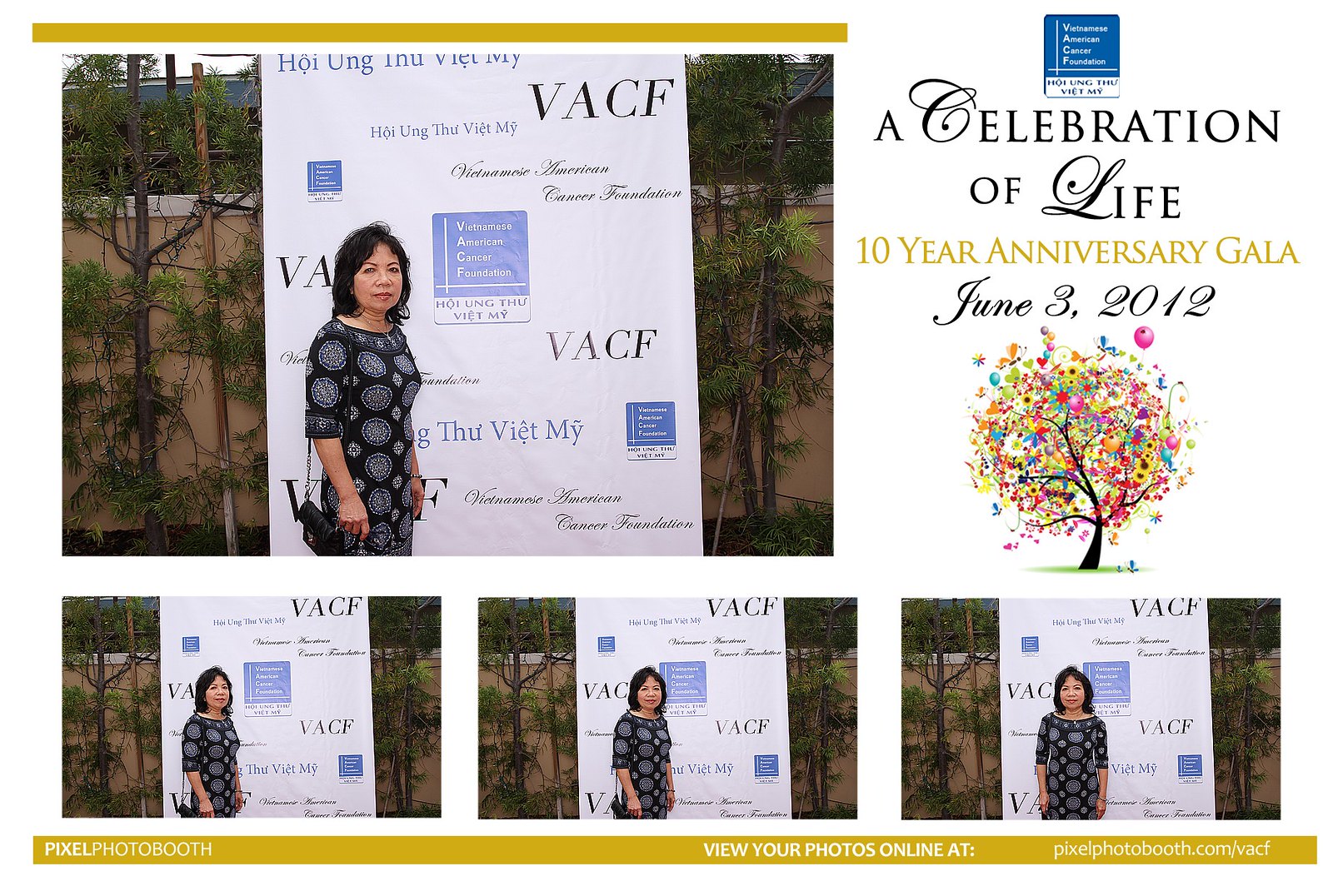The image is a montage featuring an Asian woman standing in front of a white and blue backdrop associated with the Vietnamese American Cancer Foundation (VACF). This backdrop prominently displays the VACF name and logo along with a colorful illustration of a tree adorned with various bright designs such as balloons, flowers, butterflies, hearts, and leaves. The text "A Celebration of Life: 10-Year Anniversary Gala, June 3, 2012" is visible in the top right corner. In the montage, the woman, who has shoulder-length black hair, is seen in multiple poses. She is wearing a black dress with white circular patterns and carrying a black shoulder bag. Below her images, there's a note indicating that photos can be viewed online at pixelphotobooth.com/vacf, suggesting that the event was held in a photo booth setting, where guests could take pictures and later purchase them online.